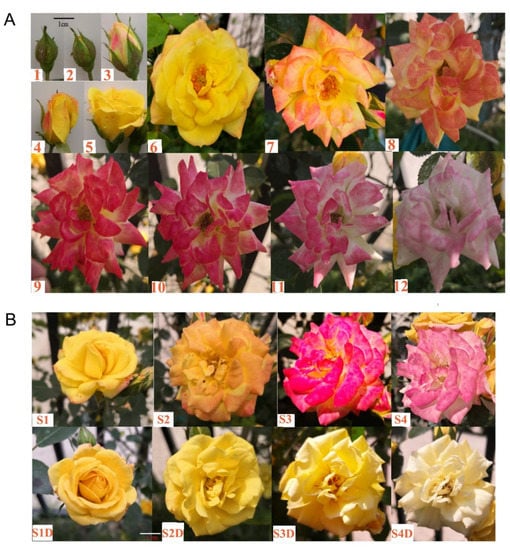The image is a high-quality, detailed diagram of various colored roses, illustrating different stages of blooming. It comprises two close-up photographs labeled 'A' and 'B' in the top left corners, with each photograph featuring eight different roses, arranged in four columns and two rows. The roses display a range of colors, including yellow, yellow-orange, orange-ish red, pinkish red, pinkish white, and almost white, all set against a green background showing some leaves and stems. The upper left photograph (Set A) visually documents a single rose bud progressing through five stages of opening, followed by three fully bloomed stages. The lower photograph (Set B) similarly showcases a variety of roses in different colors and stages of blooming, with numerical labels from 1 to 12 and additional labels s1 through s4 and s1d through s4d, adding a structured, informational element to the diagram. There is no additional text, emphasizing the visual storytelling of the rose's blooming process.